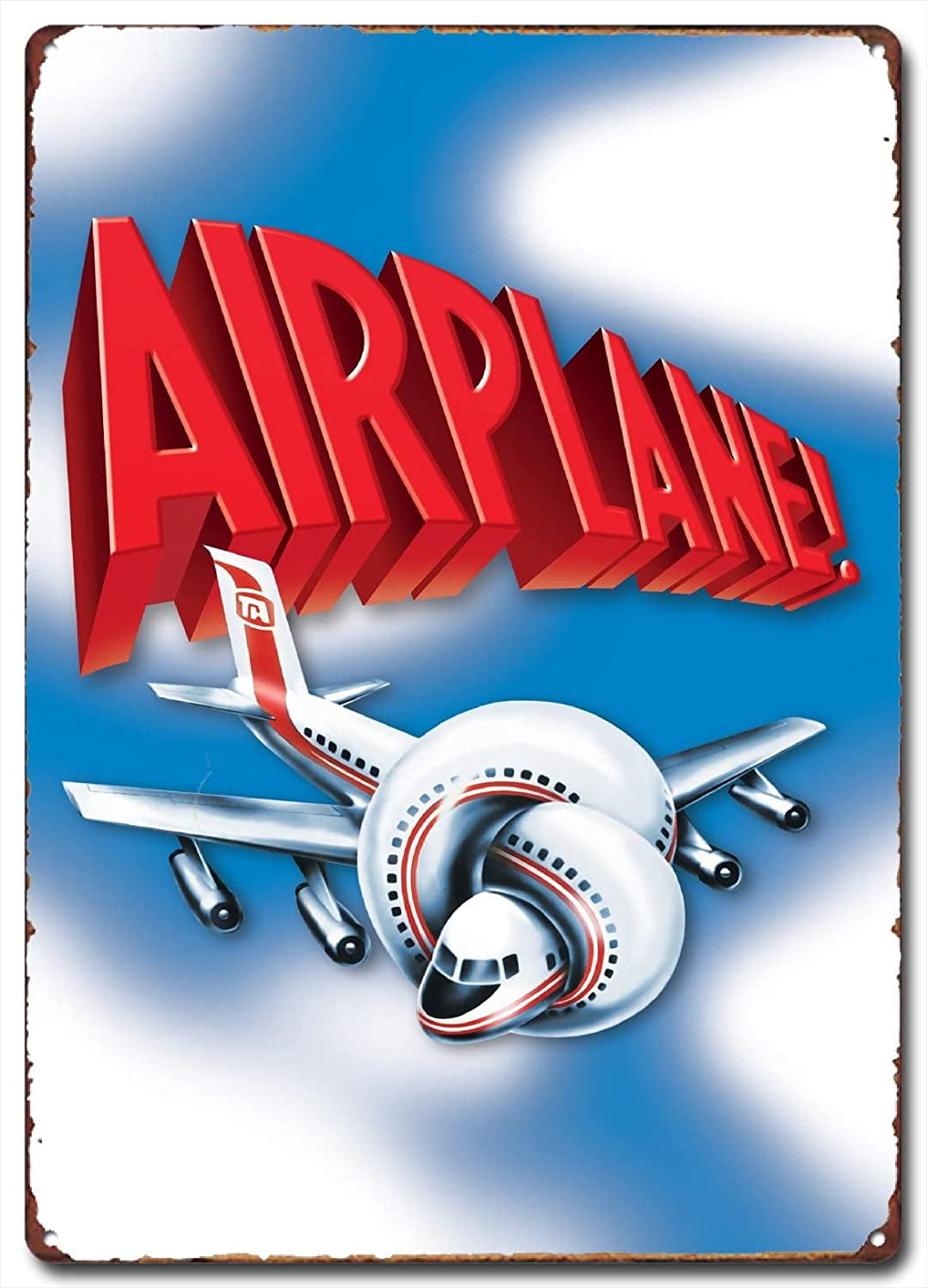This image on a rusted, rectangular metal plate—with rounded corners—features an airbrushed background of a bright blue sky dotted with soft white clouds. Prominently, it displays the word "Airplane!!!" in three-dimensional, bright red letters that start largest on the left and diminish in size towards the right, embellished with white highlights and shadowing. Below, a white passenger jet with red stripes running beneath its windows and two engines on each wing is twisted like a pretzel, its front end knotted. The tail of the plane, marked "TA," starts from the bottom of the letter 'A' in "Airplane." The sign bears the marks of time with rusted edges, adding to its character, and reflects a cartoon-like style reminiscent of the movie "Airplane."